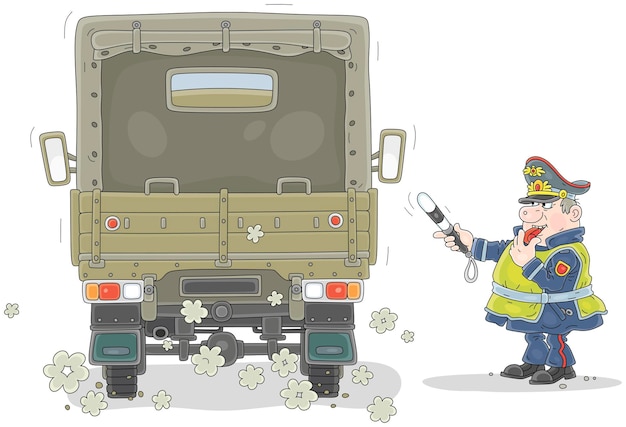This cartoon illustration presents a scene with a truck and a traffic warden set against a white background. The truck, which resembles a military vehicle with its wooden bed and brown fold-out tarp frame, is driving away, kicking up little clouds of gray and brown dust. Notably, the tarp at the back is rolled up, revealing an empty interior. The truck is detailed with rear indicators, lights in red, white, and orange, a tail hitch, black tires, and light green mud flaps.

To the right of the truck stands a traffic warden, who might be mistaken for a policeman due to his uniform. He is wearing a blue uniform topped with a peaked cap and a reflective yellow vest. In his right hand, he waves a black and white baton, signaling at the truck. A red whistle is held in his mouth, ready to be blown. The illustration also features a gray shadow below the characters, adding definition to the ground.